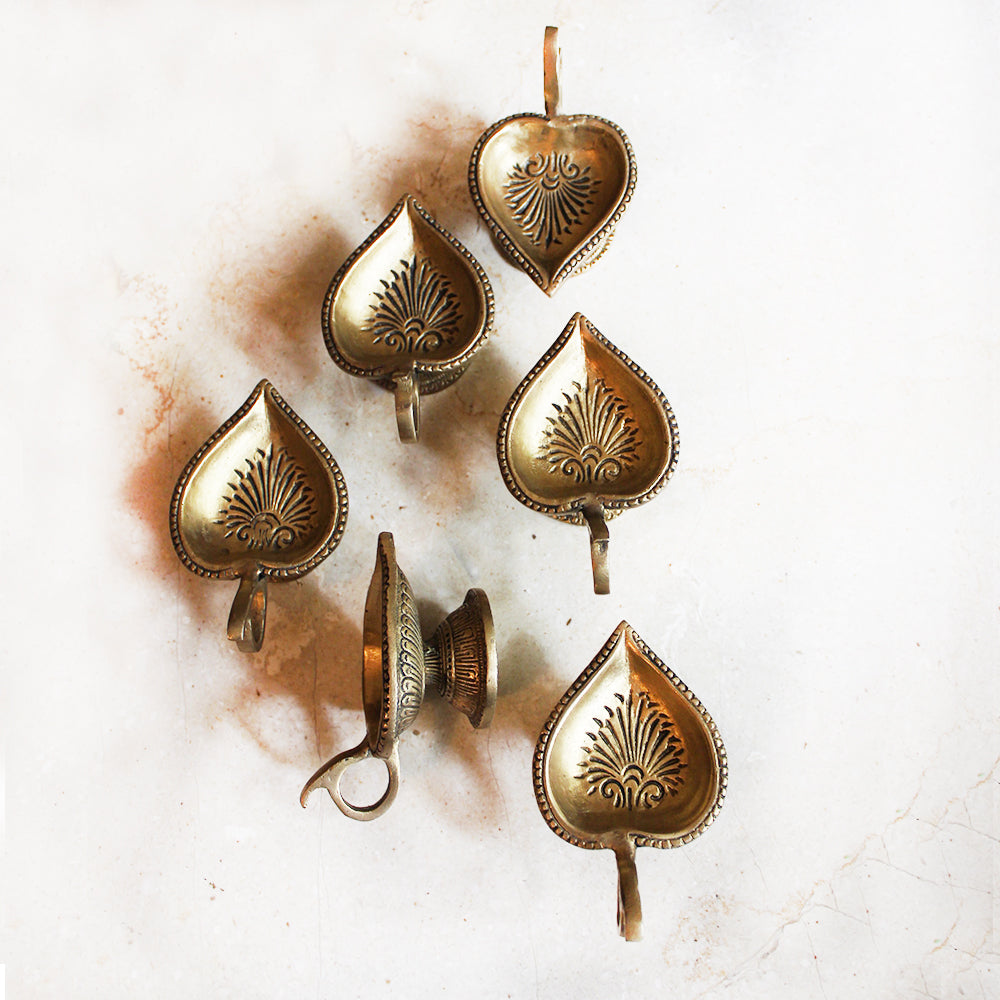This detailed illustration in portrait orientation showcases a set of six ornate, leaf-shaped serving dishes, resembling trinket or gravy trays, all uniformly colored in a bronze or brass tone. Each dish features an elaborate central engraving and a distinct handle on one side, designed to hold or pour. Five of these dishes are positioned upright, highlighting their symmetrical bouquet-like pattern and delicate edge decorations, while one is turned on its side, providing a view of its intricate side indentations and detailed perimeter. They rest on a light beige background, which contrasts beautifully with the dark brown shadows cast by each tray, enhancing their ornate design and golden-bronze coloration. The overall shape of the trays, reminiscent of teardrops or upside-down hearts, adds to their unique and decorative appeal.